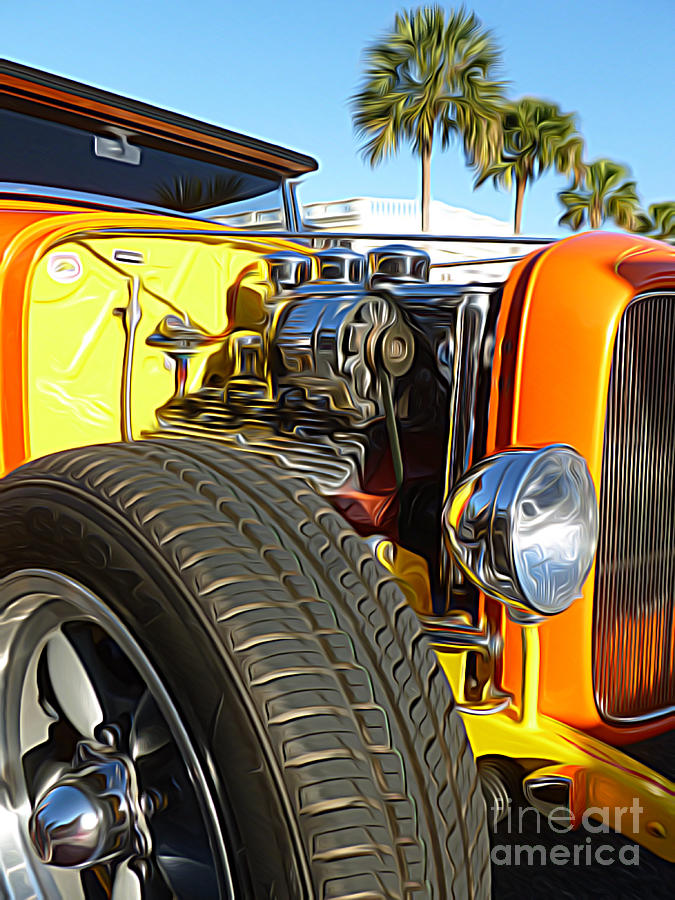The image appears to be an enhanced photograph, digitally altered with an oil paint effect, showcasing a 1932 Ford Roadster hot rod. The car, prominently positioned in the center, features an open and clean silver engine. It has an orange and yellow gradient design with modern-looking, shiny black tires and stainless steel rims. The front grill and headlight are visible on the right, while a large tire and the rearview mirror are clear in the bottom left corner. Above the windshield, the background reveals a row of palm trees against a clear blue sky and a partial view of a white building. In the bottom right corner, semi-transparent text reads "Fine Art America."